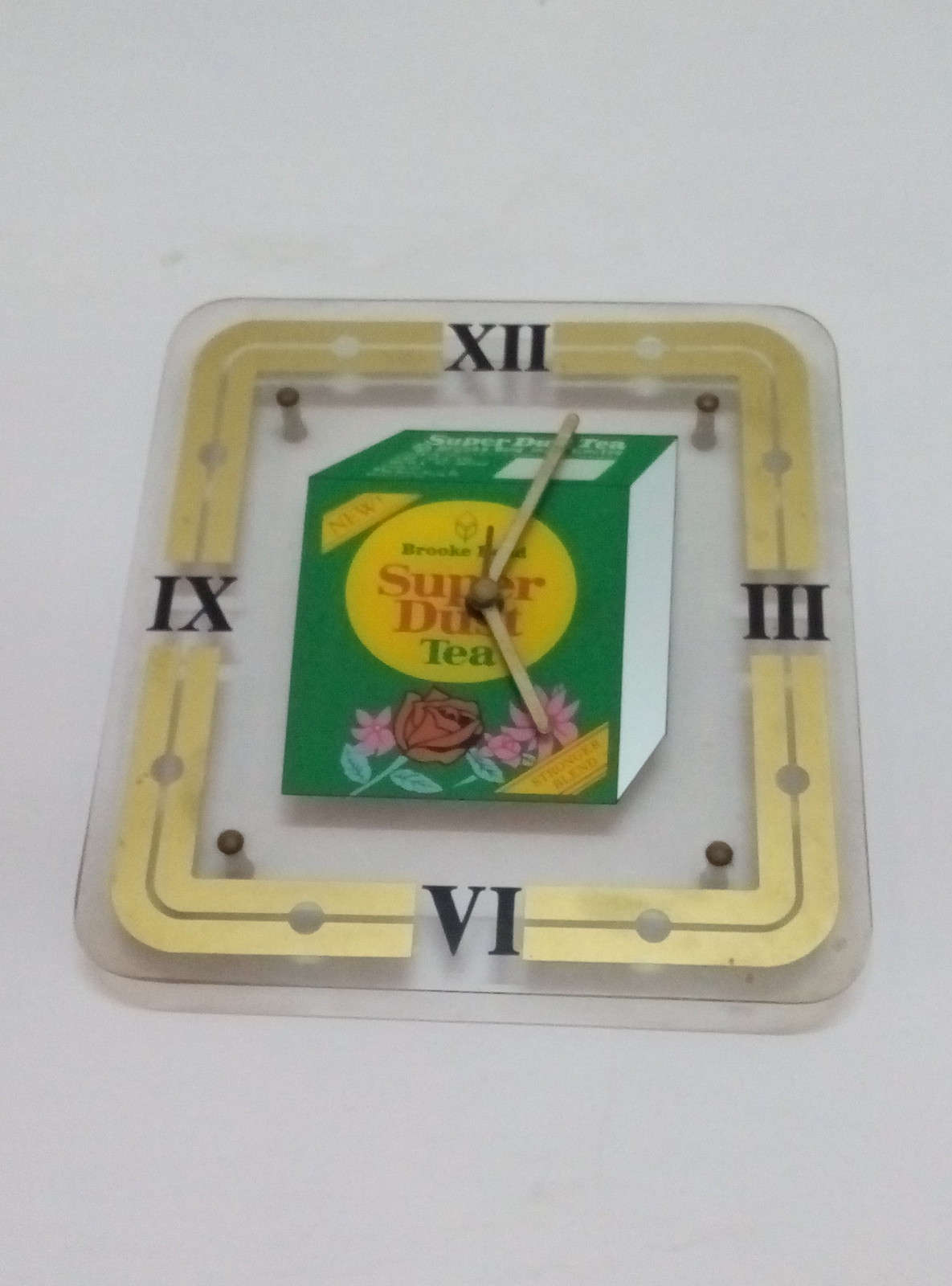In this color photograph, a distinctive clock rests on a plain white background, creating a sharp and simple contrast. The clock has a square shape with elegantly rounded edges and is framed by a double band of gold trim. Its face, made of translucent plastic or glass, showcases only the Roman numerals for 12, 3, 6, and 9. The center of the clock features an intriguing depiction of a green three-dimensional box, adorned with a circular label reading "Brooke" and, partially obscured by the clock hands, the text "Super Dust Tea." Below this, the box is embellished with stylized images of red and pink roses. The hands of the clock are positioned at approximately 5:05 p.m., intersecting the central artwork. Additionally, mounting screws are visible on the front of the clock, suggesting it could be both wall-mounted or placed on a table.